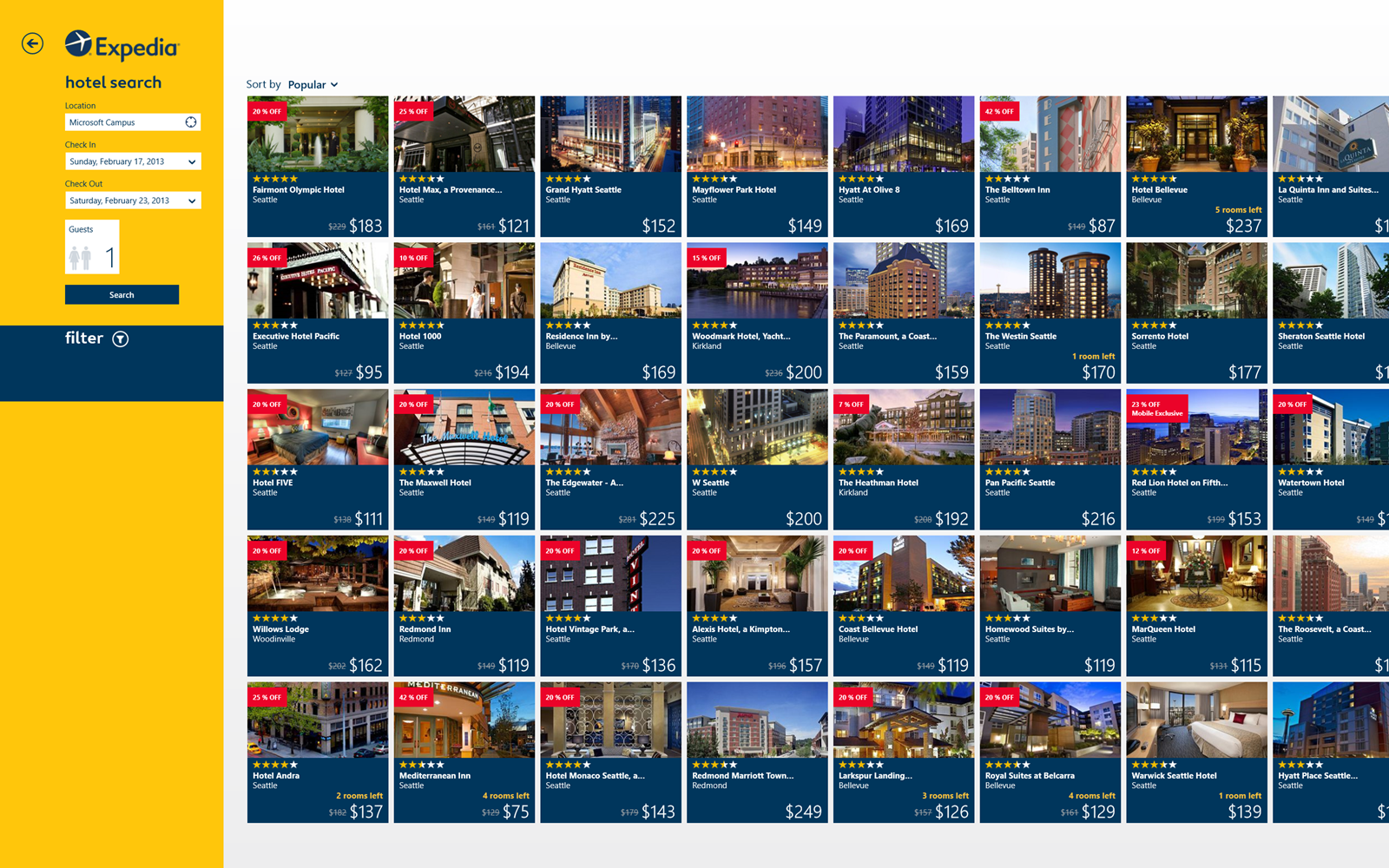The image is a square grid featuring 40 stamp-sized thumbnails of various hotels arranged in eight rows and five columns. Each thumbnail showcases either the exterior or interior of a hotel, complete with pricing information. A distinct orange bar runs vertically along the left side of the image. 

At the top of this orange bar, starting from the left, there's an arrow encased in a circle pointing to the left, followed by the Expedia icon and the word "Expedia" both in navy blue. Next to this, there's a search interface labeled "Hotel Search." This interface includes several white rectangular fields: one for entering the destination, one for the check-in date, one for the check-out date, and a square for specifying the number of guests, which defaults to one but can be adjusted. Additionally, a small blue bar labeled "Submit" is available for starting the search.

Further down, separated by a thick navy blue line, is a filter option indicated by the word "Filter" next to a downwards arrow within a circle, allowing for more specific search criteria to be applied. Many of the hotel thumbnails feature a small red square in the top left corner, likely indicating a special deal or discount.